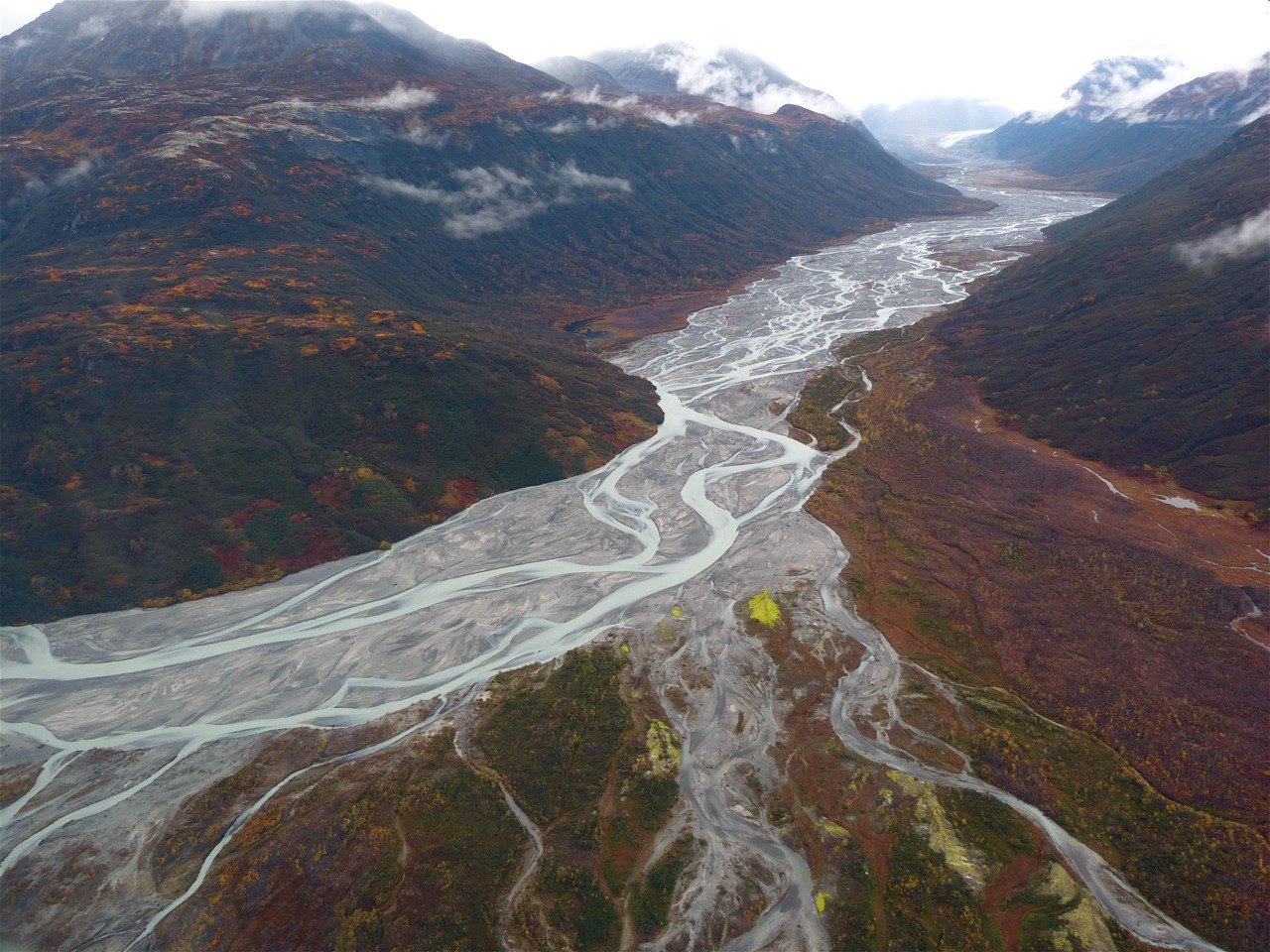This outdoor daylight photograph, taken from a high altitude, captures a striking aerial view of a glacier runoff. The image prominently features a partially frozen waterway, flowing diagonally from the upper right to the lower left. In the foreground, the rugged terrain exhibits a blend of browns, greens, and clay erosion on the valley sides, indicating prior water movement. The water not only flows but swirls, creating white streaks where the current is most active. This main stream branches off into two smaller streams towards the image's center, flowing toward the lower right corner. Surrounding the waterway, barren mountains stretch across the scene, their lower halves colored in brown and dark green, leading up to darker, nearly black peaks crowned with thin clouds. Low-lying clouds partially obscure the mountaintops in the left corner. Despite some areas blurring at the top, the realistic and vivid photograph suggests a genuine and unaltered high-altitude landscape.